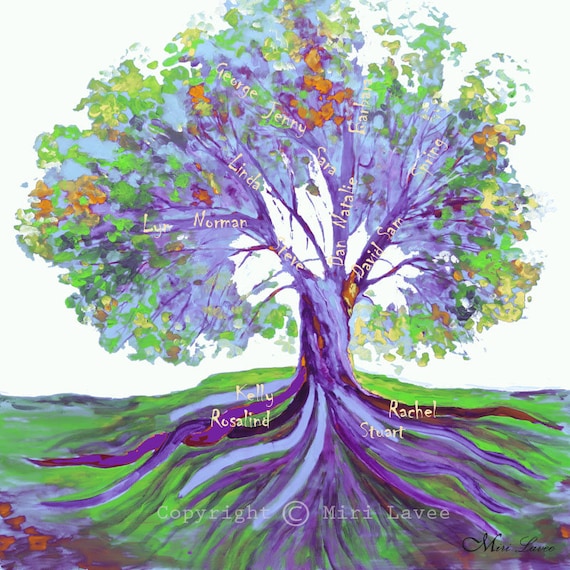This is an abstract watercolor painting by Miri Levy, as evidenced by the copyright notice at the bottom and her signature in black cursive in the bottom right corner. The painting features a surreal, vibrant tree with a robust, twisty trunk that originates from green-colored ground, suggestive of a lively landscape. The roots of the tree are depicted delicately with thin brush strokes mingling into the green field below. The tree itself is adorned with an array of colors - its branches showcase striking hues of dark blue, light blue, and various shades of purple. These branches are dotted with leaves in a kaleidoscope of green, orange, yellow, and purple tones. Among the intricate branches and leaves, numerous names are inscribed in white, including Kelly, Rachel, Rosalind, Stuart, Norman, Lee, Linda, Jenny, George, Natalie, Dan, David, Sam, Spring, and Sarah. The celestial scene unfolds against a whitish background, emphasizing the dreamlike quality of this detailed, colorful creation.